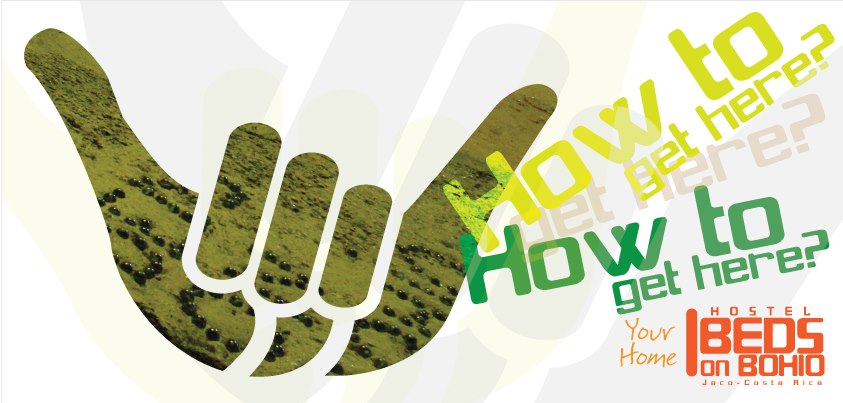This promotional poster has a clean white background and prominently features a clip art style cutout of the "shaka" sign, also known as the Hawaiian "hang loose" gesture—where the thumb and pinky are extended while the three middle fingers are folded down. This symbol is filled with a scenic greenish image that includes a field and dark colored bushes, giving it a natural look. Surrounding the graphic are gray watercolor-like shadows adding depth to the composition. 

To the right of the shaka sign, in a colorful and eye-catching arrangement, the text "how to get here?" is displayed diagonally, with the phrase repeating in various color fonts: first in yellow, then in green. Further down, "your home" is highlighted in orange, and "hostel beds on Bo-Hi-Oh" is written in a darker orange.